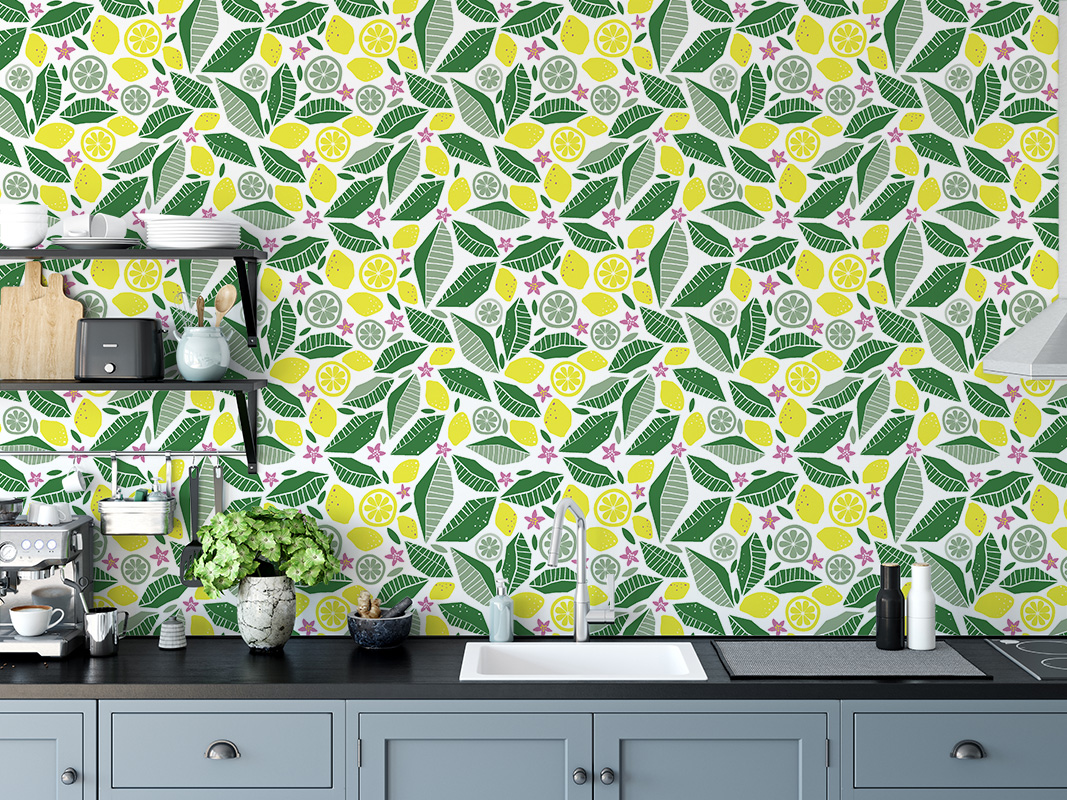The image depicts a sleek and modern kitchen counter, featuring a black surface made from what appears to be plastic or Corian material. Central to the counter is a small, stark, chrome faucet with a square, white sink. To the right of the faucet sits a pair of salt and pepper shakers designed to resemble small beer bottles—the white salt shaker on the right and the black pepper shaker on the left. The wall behind the sink is adorned with vibrant wallpaper showcasing green leaves interspersed with whole lemons, limes, and their slices. 

To the left of the sink, a structured array of kitchenware is organized on a metal shelf that holds white plates, cups, saucers, cutting boards, and a pencil holder. Below, the counter accommodates a coffee maker and a toaster, complemented by two potted plants that add a touch of greenery. Additionally, the shelves feature racks for convenient storage, and an espresso machine is prominently placed. The surrounding cabinets and drawers are presented in a clean, gray finish, adding to the organized and polished look of the kitchen. Light illuminates the scene from the left, highlighting the meticulous arrangement and modern aesthetic of the interior.